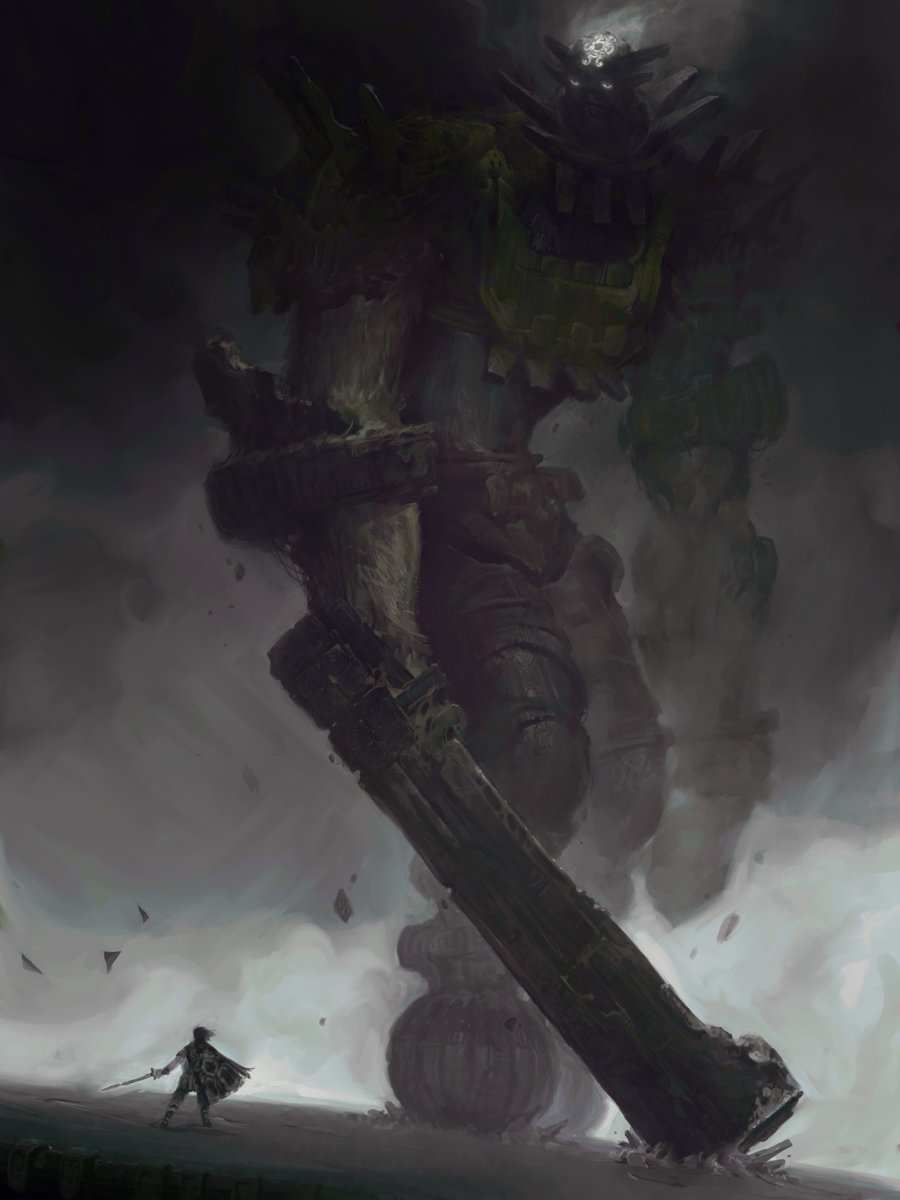In this striking painting, a colossal armored figure towers over a solitary hero positioned in the lower left-hand corner, creating a dramatic contrast between the two characters. The giant, clad in an intricate ensemble of dark blue and dark green armor, commands attention despite much of its body being obscured by the painting's deliberate use of lighting. Its chest plate showcases a compelling dark green and yellow mixture, while menacing yellow eyes with white highlights peer downwards at the hero, exuding a sense of foreboding.

A luminous area at the crest of the giant’s head radiates light upwards, piercing through the oppressive dark gray clouds and casting them into a lighter shade. Spikes adorn the giant's head and chest armor, the latter of which is a somber dark gray. Its massive arms, cloaked in dark gray and black armor that transitions to a lighter gray at the extremities, add to its menacing presence. The right arm and leg are subtly faded to enhance the three-dimensional effect of the figure’s imposing stature. 

The lower part of the giant's attire features brown leggings near the torso, blending into dark green and black armor on its left side. Clutched in its hand is a formidable black sword, accented with streaks of yellow and green, further emphasizing its intimidating nature.

Contrasting starkly with the giant, the small hero is depicted as a silhouette draped in a dark green cape embroidered with golden and yellow designs. The hero sports shoulder-length brown hair and is dressed in cloth-like armor with matching shoes. His left hand grips a sword, and he gazes resolutely upwards at the towering behemoth. The atmospheric painting also features small triangles and fragments seemingly falling from the giant, adding a dynamic sense of motion to the scene, while the ground below remains shrouded in dark gray tones.